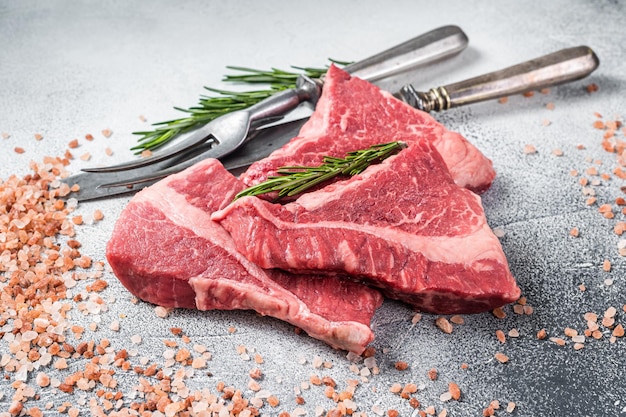This photograph features three overlapping raw steaks arranged in a small, neat pile on a gray, speckled stone surface. The rich marbling and the thick strip of white fat running through the center of the steaks emphasize their quality. Sprigs of green rosemary rest atop and beside the steaks, adding a touch of freshness to the image. An old-fashioned, patinaed two-pronged fork and a steak knife are positioned behind the meat, enhancing the rustic and professional aesthetic of the setup. Surrounding the steaks and cutlery, large grains of Himalayan pink salt are scattered, contributing both vibrant color and a hint of seasoning to the composition. The photograph, well-lit and likely professional, showcases a meticulous and appetizing presentation of the raw steaks on the gray stone-like surface.